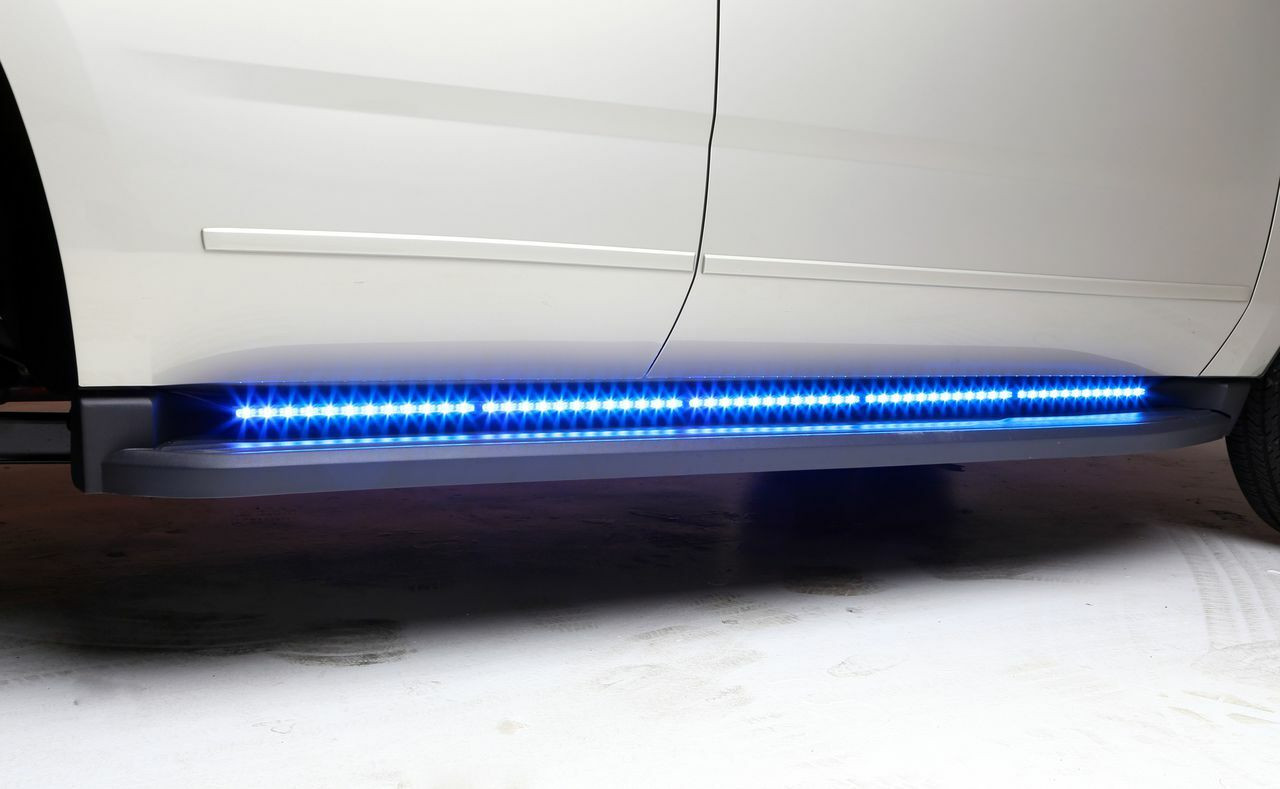The image features a detailed close-up of a clean, white vehicle parked in an area with a white-painted concrete floor, which has visible black tire marks. The focus is on a gray step board running beneath the driver's side and rear driver's side passenger doors. Above the step board, a line of bright blue, segmented LED lights illuminates the area, drawing attention to the footstep used for entering the vehicle. The image is taken from a zoomed-in perspective, emphasizing the LED lights, but also capturing the lower part of the car's clean white doors with some molding detail and a glimpse of the rear tire. The vehicle appears to be relatively low to the ground, suggesting it could be an SUV or a car, and the scene is set in a garage-like space.